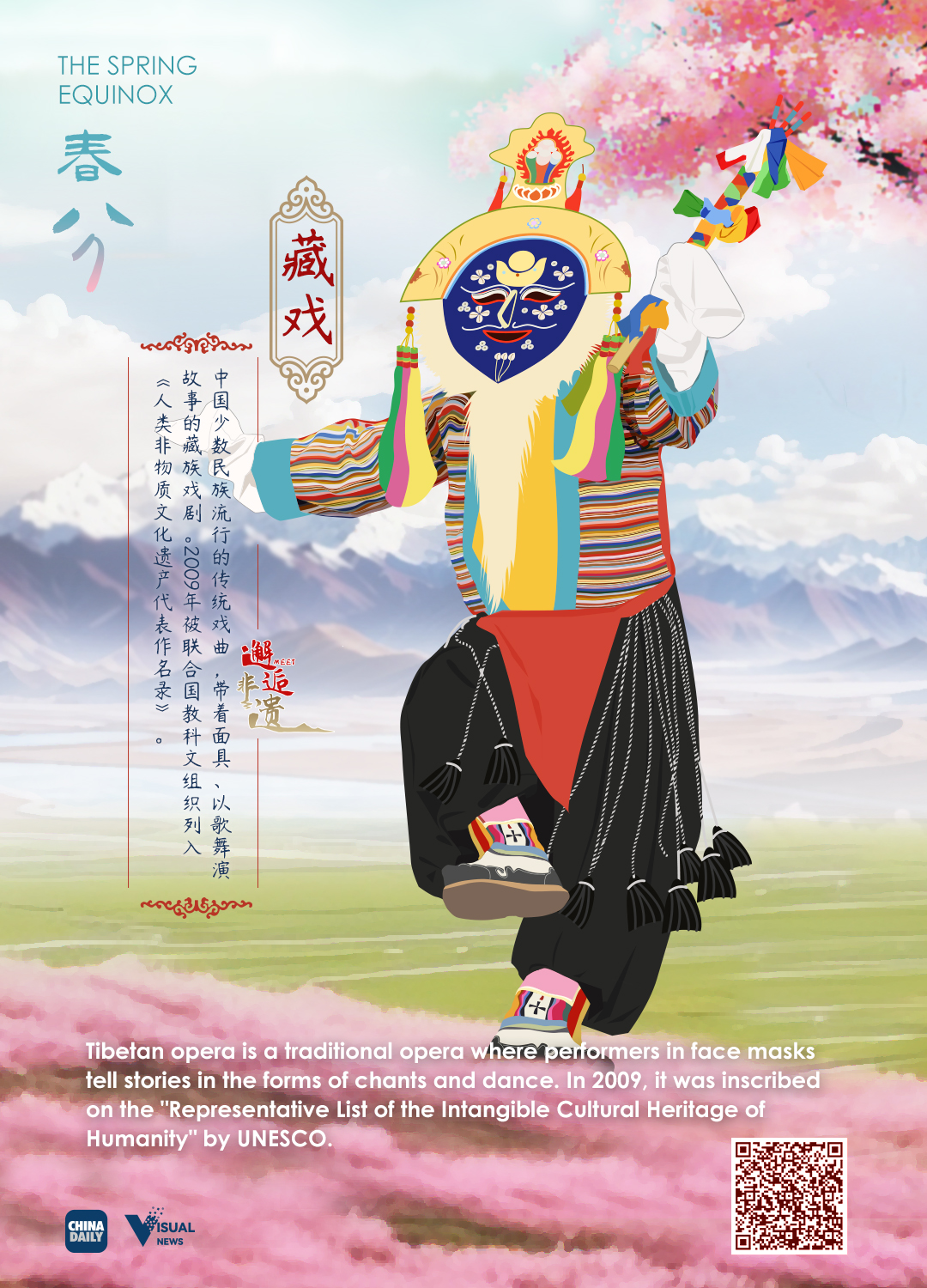The image is a computer-generated heritage illustration that features a character in traditional Tibetan opera costume. This character is wearing a blue mask adorned with a gold arc on the top and yellow hairs at the bottom, along with black pants and some red detailing. The backdrop showcases a serene setting with a blue sky and white clouds. The illustration includes numerous Asian characters, with significant text on the left, including a title at the upper left that reads "Spring Equinox," likely indicating the theme of the dance. At the bottom of the image, there's a descriptive paragraph explaining that Tibetan opera is a traditional form of opera where performers in face masks tell stories through chants and dance. This form of opera was inscribed on UNESCO's representative list of the intangible cultural heritage of humanity in 2009. In the bottom right corner, there's a QR code, and in the bottom left, the text "China Daily" and "Visual News" is visible. The image is also accented with pink at the bottom.